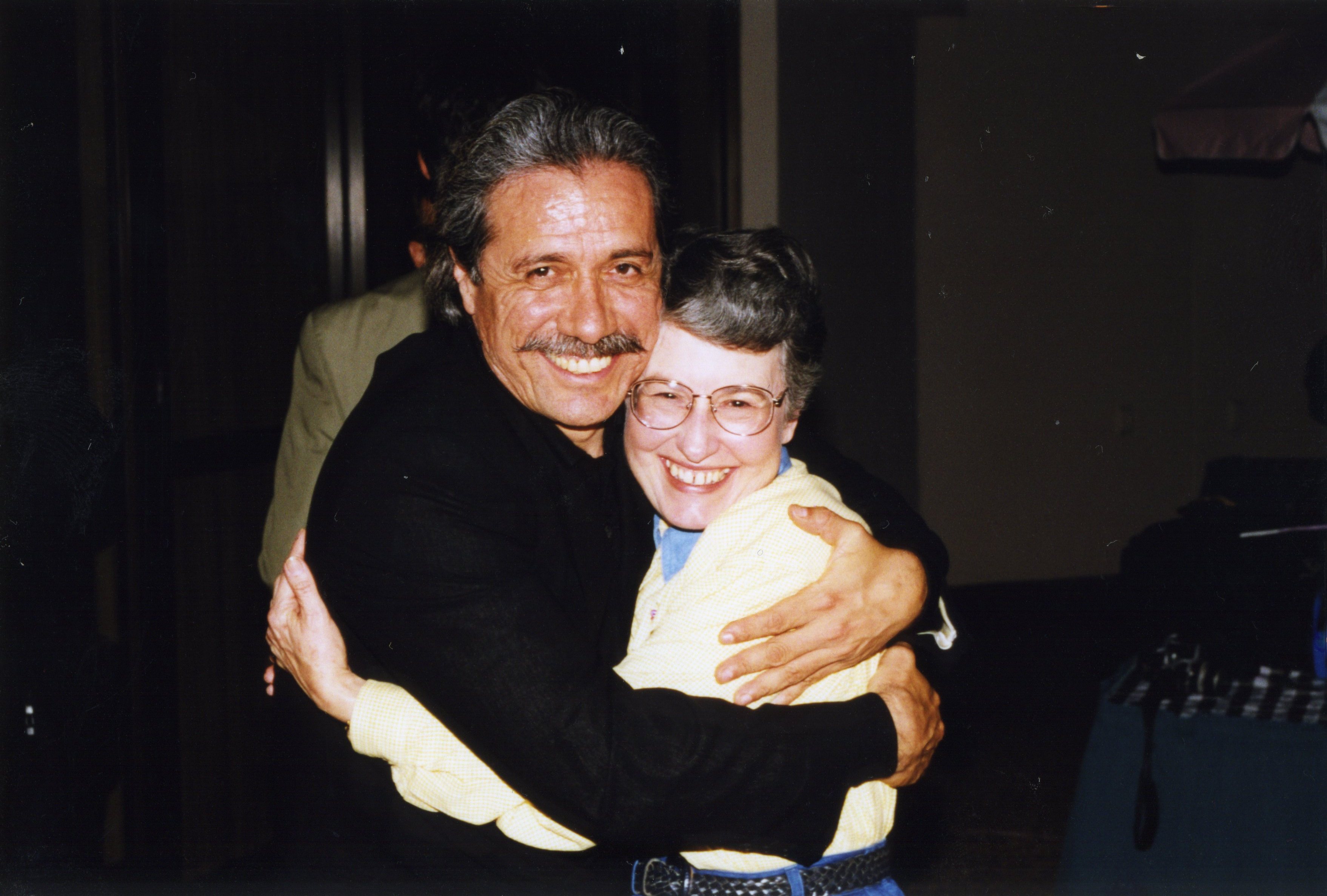The photograph captures an intimate and joyful moment between two older adults who are warmly embracing each other and beaming directly at the camera. The man on the left has gray and black hair slicked back, complemented by a gray mustache. He is dressed in a black coat paired with a black shirt and is smiling broadly, revealing his upper teeth. The woman on the right sports a short bob haircut with dark hair flecked with gray. She is wearing gold-rimmed glasses and a yellow button-up shirt with a blue collar, tucked into blue jeans, completed with a black braided leather belt featuring a silver buckle. Her radiant smile also reveals her upper teeth. Given their clothing and the presence of a flash highlighted against the dark backdrop, it appears they are indoors at an event, possibly in a hotel lobby or similar venue. Their arms encircle each other, capturing a sense of warmth, happiness, and connection.